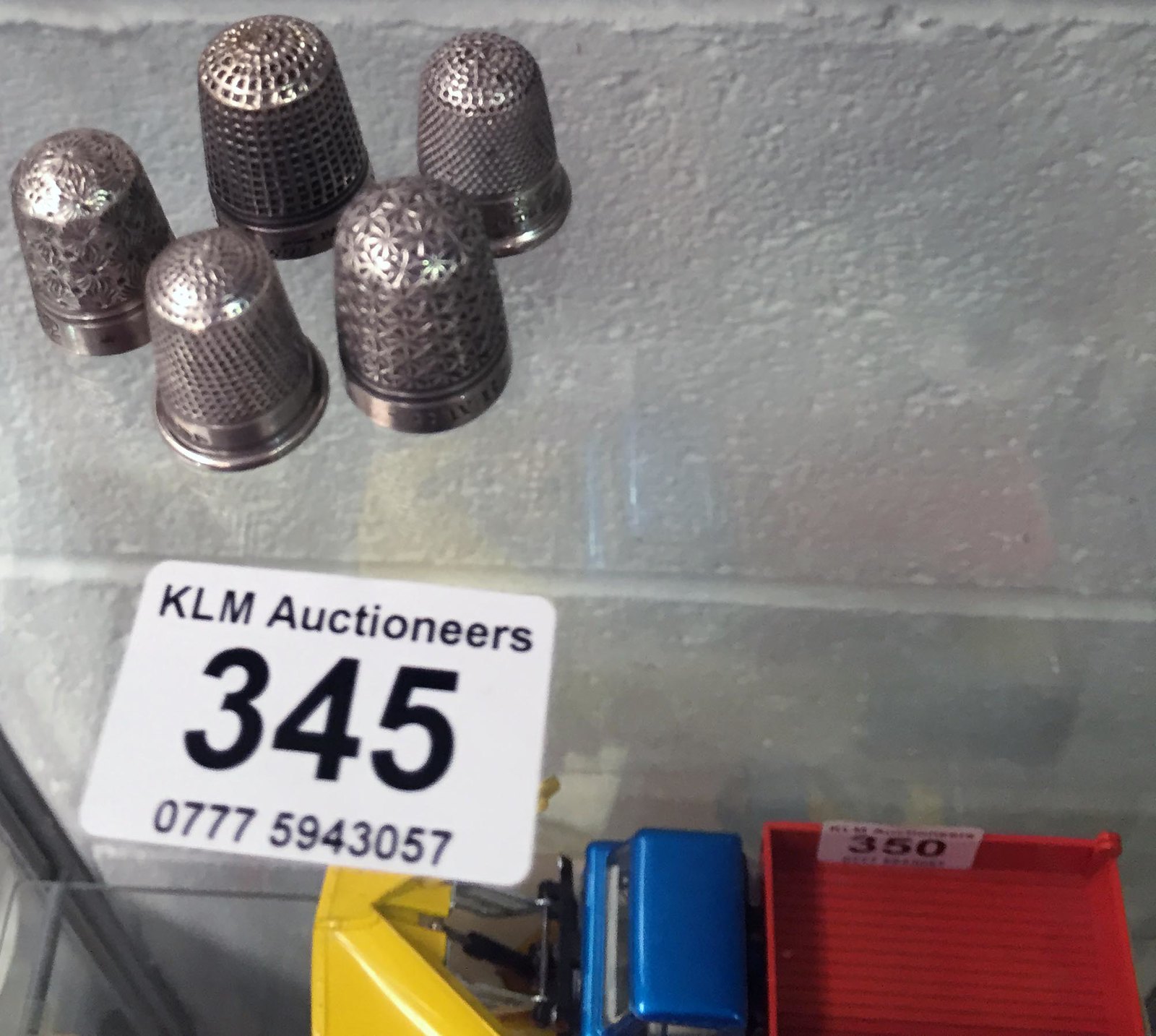This detailed photograph, taken inside an auction house, showcases a display case featuring five silver thimbles with various intricate indentations and patterns on their metal surfaces. The thimbles, each unique in design—one with a basket weave pattern, another dotted, and some featuring deeper indentations on their tops—are neatly arranged on a glass shelf against a backdrop of rough, white-painted cinder block walls. A white sticker affixed to the shelf reads in black text: "KLM Auctioneers," followed by the number "345" and a serial number "0777-594-3057" beneath it. Below this shelf, a hint of a second shelf is visible, containing a few indiscernible items, including a notably vivid yellow object, a blue object potentially resembling a toy truck with a red tipper, and a red bin marked "350" on a white label. The scene elegantly captures a moment within the auction environment, emphasizing the displayed thimbles and the other intriguing items below.